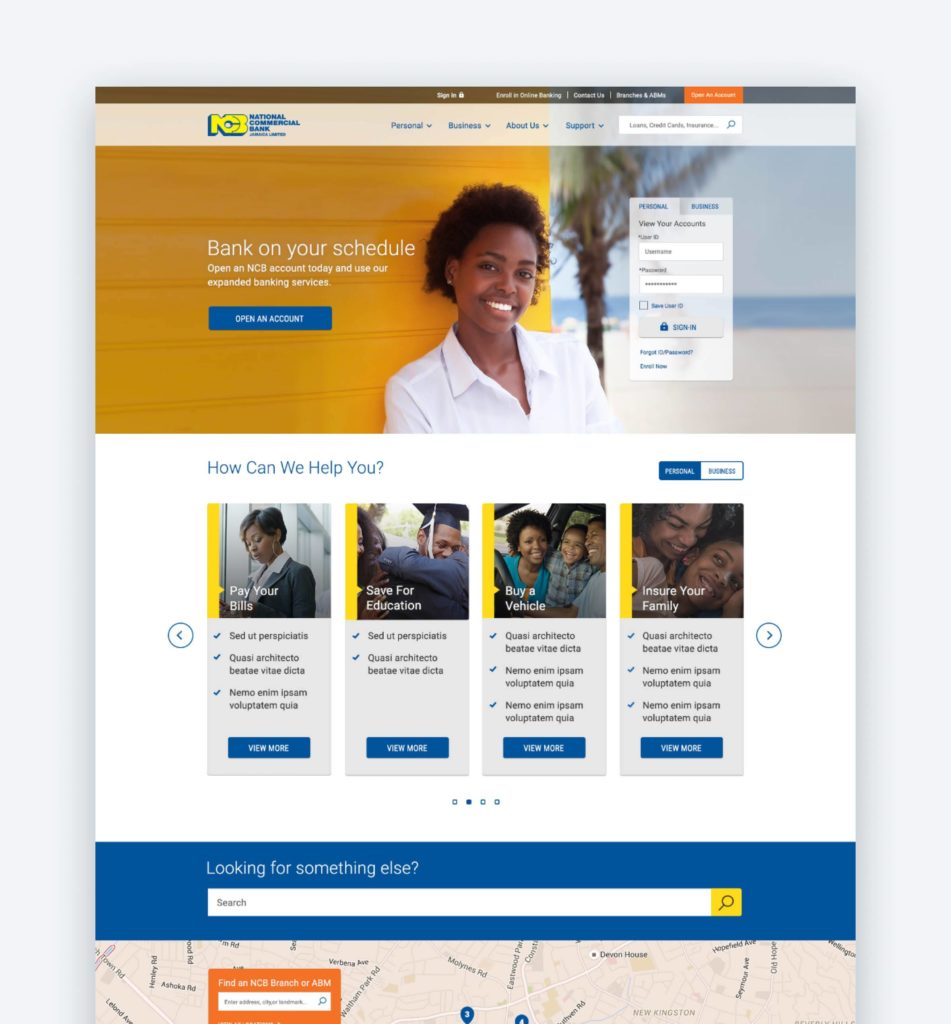Screenshot of the National Commercial Bank Website:

The top of the screen features a large horizontal banner that dominates the webpage, showcasing a vibrant photo. At the center of the image, a woman with short, dark hair and dark skin leans casually against a yellow wall adorned with horizontal plank-like paneling. Her relaxed pose contrasts with her crisp, white shirt, which slightly wrinkled, hints at a leisurely yet professional demeanor. She gazes directly at the camera with a gentle tilt of her head to the right while her body angles to the left.

To the right of the woman, the scene transitions into a stunning beach panorama, complete with pristine white sand, a sparkling blue ocean, and a palm tree, slightly out of focus at the top, adding a touch of tropical charm to the composition. The peaceful beach setting juxtaposes seamlessly with the professional appeal of the woman, conveying a balanced lifestyle message.

Superimposed on the yellow paneling beside the woman, bold white text reads: “Bank on Your Schedule. Open an NCB account today and use your expanded banking services.” Beneath this compelling call-to-action, a prominent blue rectangular button invites viewers to “Open an Account,” encouraging engagement with the bank’s services.